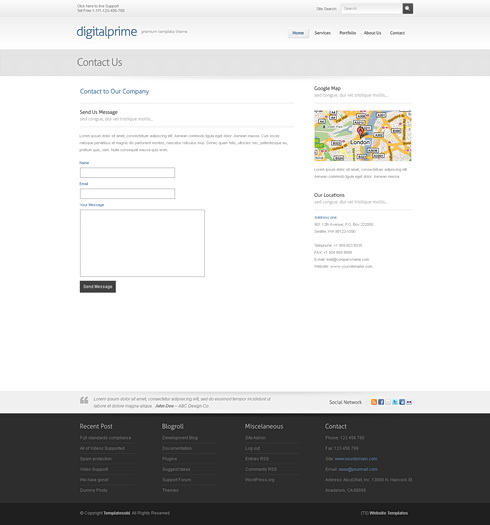This image depicts a somewhat out-of-focus web page, making some of the text difficult to read. In the top left corner, there's a clickable link for live support and a toll-free number, though the phone number itself is blurry and illegible. The top right corner features a "Search" function with a search box next to it. 

Below these elements, in larger, bold text, the word "DigitalPrime" is displayed, followed by more illegible text. As you scan across the page, the navigation bar lists sections such as "Services," "Portfolio," "About Us," and "Contact."

Lower on the page, under the enlarged heading "Contact Us," there is an invitation to reach out to the company, with prompts like "Contact our company, send us a message." Beneath this, the remaining text is blurry and appears to be in a foreign language. 

Further down, there are labeled fields for "Name" with an empty input box, "Email" followed by another empty input box, and "Message" accompanied by a larger, empty text box. At the bottom of this section is a black button labeled "Send Message."

On the far-right side of the page, there's a header that says "Google Map" showing a map with "London" as the central label. Various parts of the map are highlighted in yellow. Below the map, the section titled "Our Locations" lists a couple of locations, though this text is also blurry and difficult to decipher.